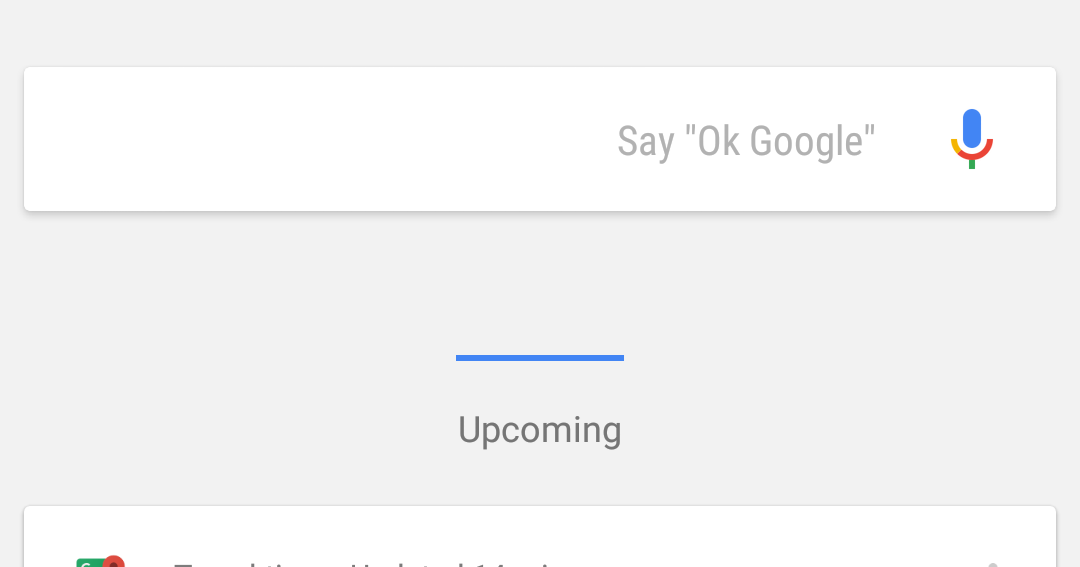The image displays a Google search interface with a primary focus on the voice search option. Dominating the frame is a search bar that reads "Hey Google" or "Say OK Google," accompanied by a white rectangular button that spans the full width of the interface. To the right of this button is a prominent blue microphone icon. 

Below the search bar, a centered blue line serves as a separator. Directly beneath this divider, it says "Upcoming" in black text, indicating a new section. This "Upcoming" text marks the beginning of a new box, which also has a white background. However, the text within this section is difficult to discern, though the layout resembles the upper part of the Google Maps app, with some indistinct writing.

The backdrop of the entire interface is a light gray, contrasting with the highlighted areas of white and blue. The functionality of the microphone icon is to enable voice input, allowing users to speak their queries instead of typing them, offering a convenient alternative for those who find verbal communication quicker or easier than typing.